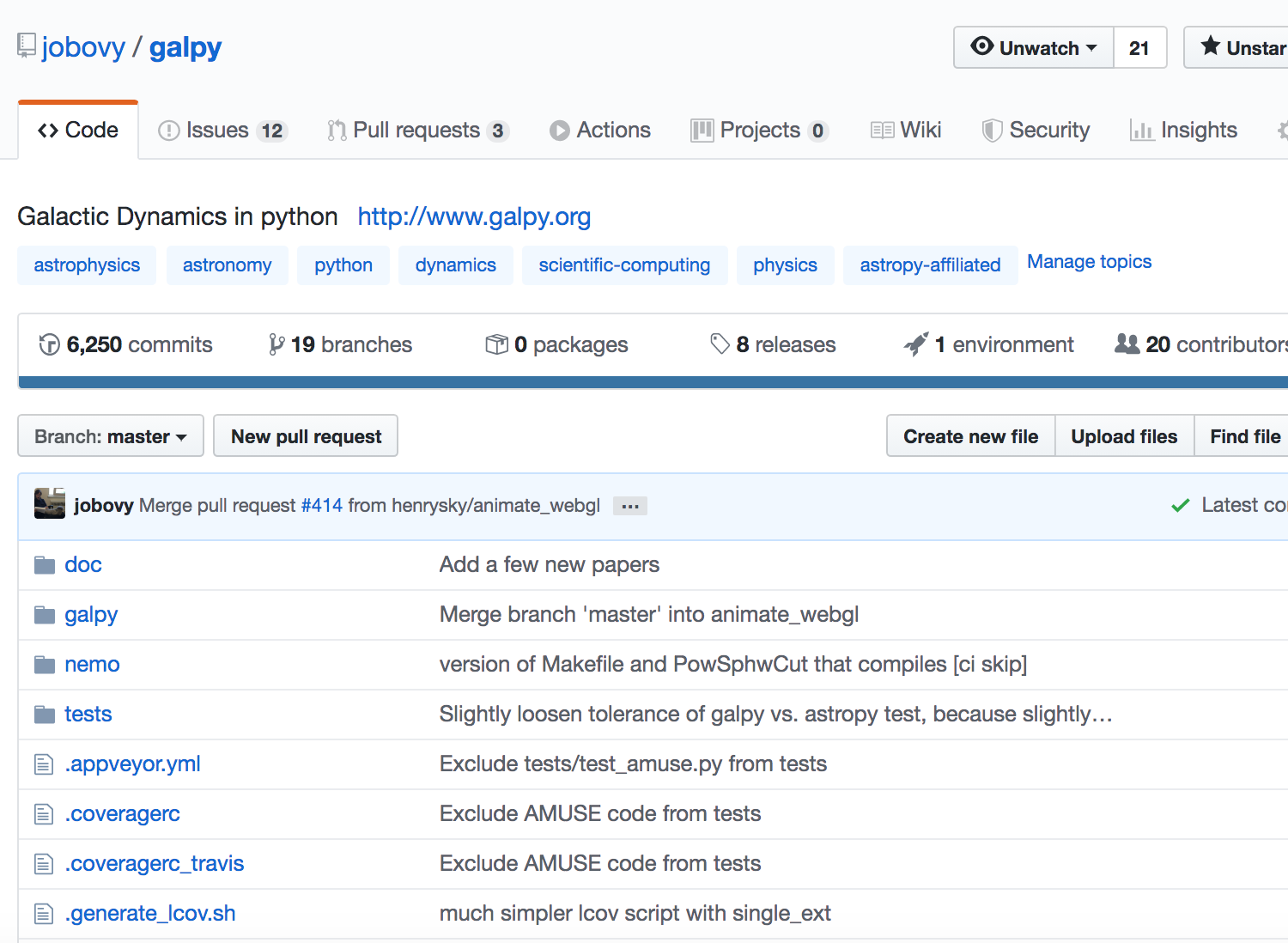This screenshot captures a web page showcasing a detailed user interface, primarily focused on a project repository or similar content management system. 

At the very top, a light grey header spans the width of the page. Situated on the top left of this header is a medium grey icon depicting a book with a bookmark protruding from the bottom. Adjacent to the icon, thin blue text reads "Jabovi," followed by a black slash and bold blue text that says "Galpi."

Directly below this header, a navigation tab is prominently selected. This active tab is white with an orange line across the top, indicating its selection. Within this tab, black text reads "Code," flanked by black arrow brackets facing left and right respectively.

To the right of the active "Code" tab, there are additional tabs each labeled with dark grey text and accompanied by various icons. The sequence of these tabs is as follows:

1. **Issues:** Featuring a light grey exclamation point icon enclosed in a light grey circle outline to the left, and a light grey oval with the black number "12" to the right.
2. **Pull Requests:** With a unique icon to the left, consisting of a vertical medium grey line and a twisted medium grey arrow pointing left. Both the line and the arrow are capped with medium grey circle outlines. A light grey oval with the black numeral "3" accompanies this tab on the right.
3. **Actions:** Displaying a medium grey circle with a light grey triangle pointing right within it.
4. **Projects**
5. **Wiki**
6. **Security**
7. **Insights**

Each element and icon is distinctly designed to provide a clean and organized navigational experience, enhancing the user’s ability to manage and access various features within the repository efficiently.